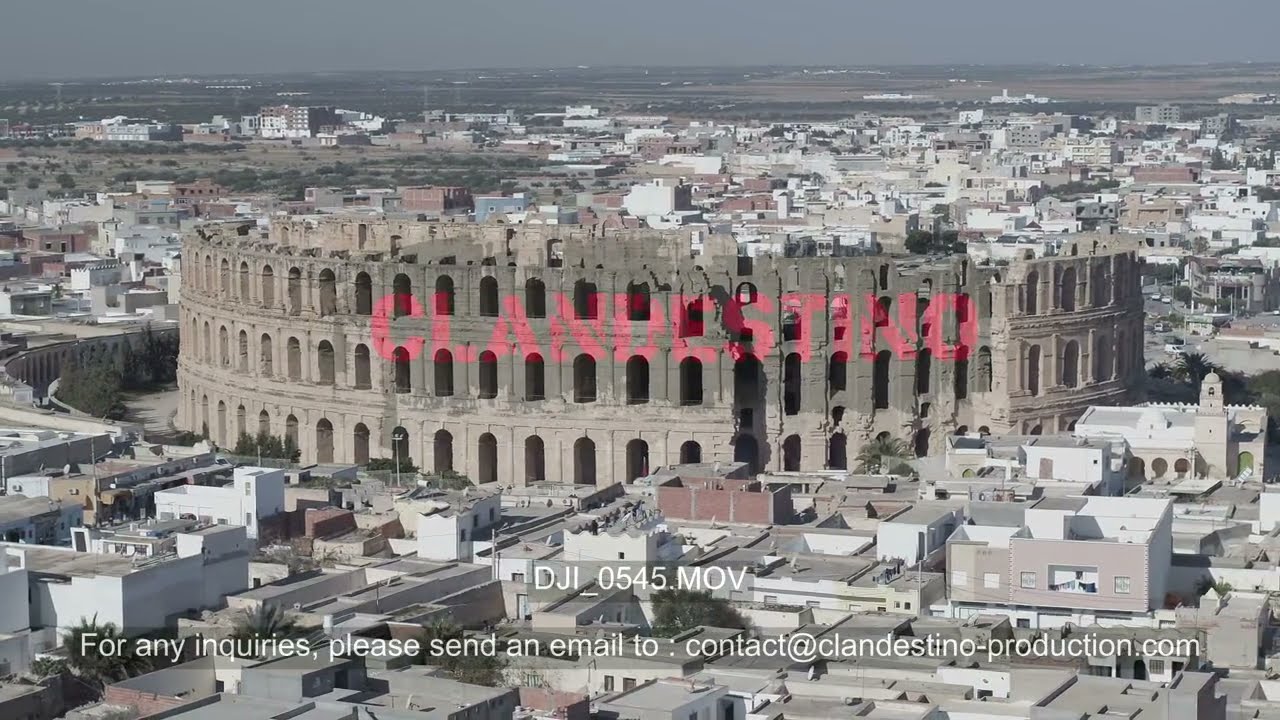The image is a wide rectangular photograph capturing a high, slightly overhead view of an ancient three-story Colosseum, centrally placed in the middle of a bustling cityscape. The Colosseum's exterior is constructed of light brown bricks, each level adorned with curved rectangular windows. Surrounding the historic structure is a mix of shorter buildings painted in various hues—reddish-brown, white, gray, and tan—forming a vibrant urban backdrop both in front of and behind the monument. 

At the outskirts of the cityscape, the scene transitions into a more rural setting, with green farmland and lengthy roads dotted with vehicles extending into the distance. The city streets appear devoid of visible people or heavy traffic, focusing attention on the architectural elements. 

The image contains several overlaid texts: "clandestino" is prominently displayed in transparent red on the Colosseum, and at the bottom, it reads "Capitols" in white and "DJI_05.45.MOV," suggesting the image might be a still from a video. Additionally, a note for contact reads, "For any inquiries, please send an email to contact@clandestinoproduction.com."